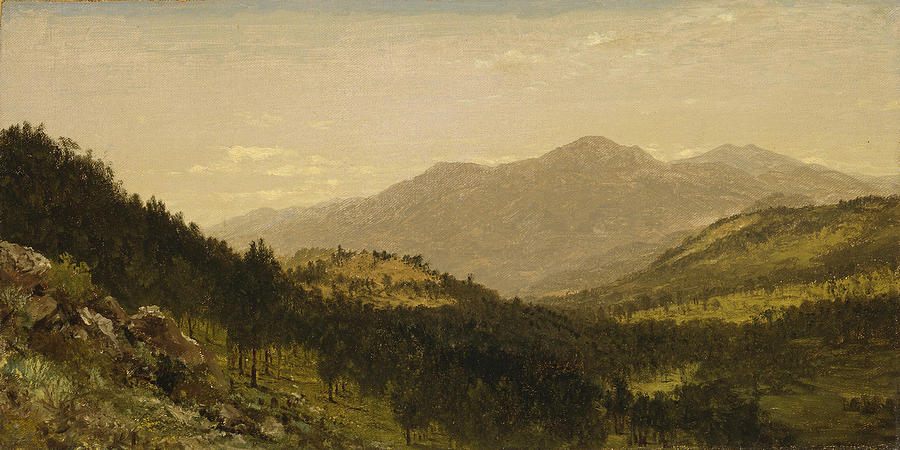The painting depicts a tranquil valley set in a mountainous region. Leading from the foreground to the background, the scene transitions from scattered rocks and shrubbery to a richly forested area, culminating in a rugged mountain range with several peaks shaded in brown. The trees, in various shades of dark and light green, have brown trunks and dot the landscape, creating a lush canopy. The sky overhead is a light gray, possibly hinting at dawn or dusk. Prominent in the foreground on the left are detailed rocky formations, while trees stretch across the upper left part of the painting and down into the valley, continuing to the right until they meet the mountains. Small huts are subtly nestled among the trees, adding a touch of human presence to the otherwise wild and verdant scenery.